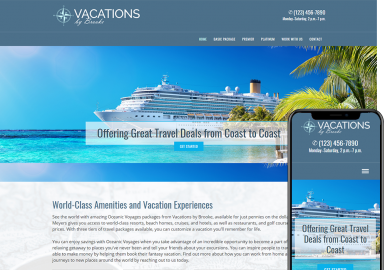The image is a low-resolution advertisement for vacation cruises. The top section features a light blue background with the word "Vacations" in cursive text alongside a compass symbol, indicating the archival header. A phone number is also present but unreadable due to the resolution.

In the center of the image, there is an expansive cruise ship extending from the right side of the frame, surrounded by clear, blue skies and palm trees in the background, creating a picturesque tropical setting. Overlaying the image of the cruise ship is a white box with the promotional text, "Offering great travel deals from coast to coast."

At the bottom right, a smartphone display mirrors the website's layout, including another visible phone number and identical promotional text. The smartphone screen shows a white border at its bottom with dark blue text stating, "World-class amenities and vacation experiences." Below this header, there are two paragraphs of gray text, which are illegible due to the image's resolution.

Overall, the advertisement is visually centered around the cruise ship, emphasizing enticing coastal vacation packages and luxurious travel experiences.